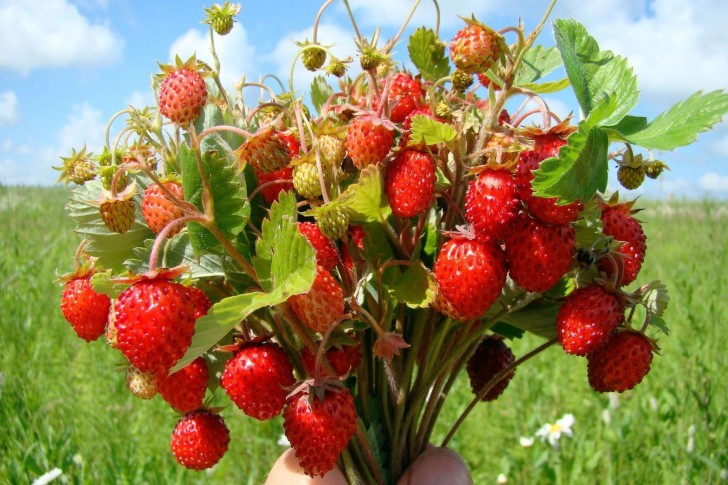In this detailed photograph, a person is holding a large, vibrant bouquet of strawberries, prominently featuring an array of strawberries in various stages of ripeness. At the forefront are the ripe, plump, and bright red strawberries, which almost resemble flowers with their vivid color and lush appearance. Intermixed among the ripe berries are some smaller, green strawberries that have not yet ripened, as well as ones that are transitioning from pink to red, still displaying streaks of green. Scattered throughout the bouquet, there are also buds where strawberries have yet to fully develop.

The strawberries are attached to notably long stems, which is unusual compared to the shorter stems typically seen in stores, and these stems are clasped by a hand at the bottom of the image. Surrounding the strawberries are their green leaves, adding to the bouquet-like aesthetic. 

In the background, a picturesque scene unfolds with a grassy field dotted with white and yellow daisies, under a clear blue sky adorned with large, fluffy white clouds. This serene setting, combined with the colorful array of strawberries, creates a striking and harmonious composition.